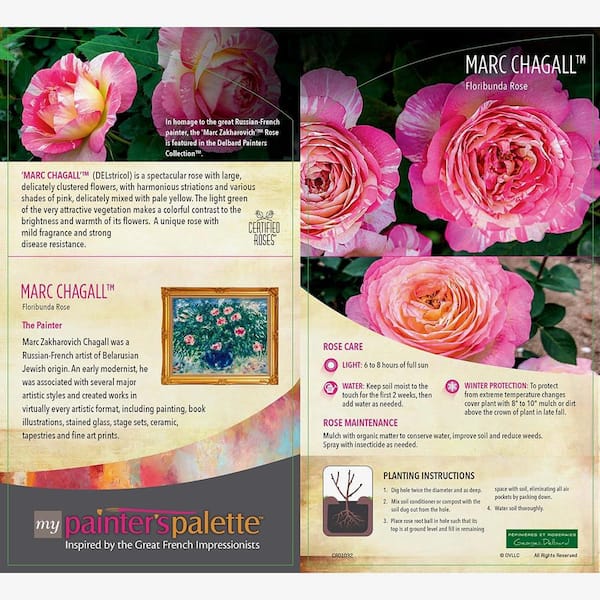The image displays a two-page spread from a pamphlet or magazine, predominantly showcasing pink and white floribunda roses. The background is a mix of brown with various black, red, and green highlights. On the left page, at the bottom corner, the text "My Painter's Palette" is prominently featured, with "painter’s" in pink, "palette" in orange, and "my" in white. Below it, in white lettering, reads "Inspired by the great French impressionists," alongside a reference to the painter Mark Chagall, with a paragraph discussing his significance.

The top section of the left page zooms in on the fully bloomed roses with lush green foliage, creating a striking visual. The right page is dedicated to detailed care instructions for the floribunda roses, titled "Mark Chagall Floribunda Rose." This section provides guidance on lighting (6-8 hours of full sun), watering, winter protection, and overall maintenance. The text related to rose care and planting is written in pink, and the informative layout is neatly organized for easy understanding of each step.